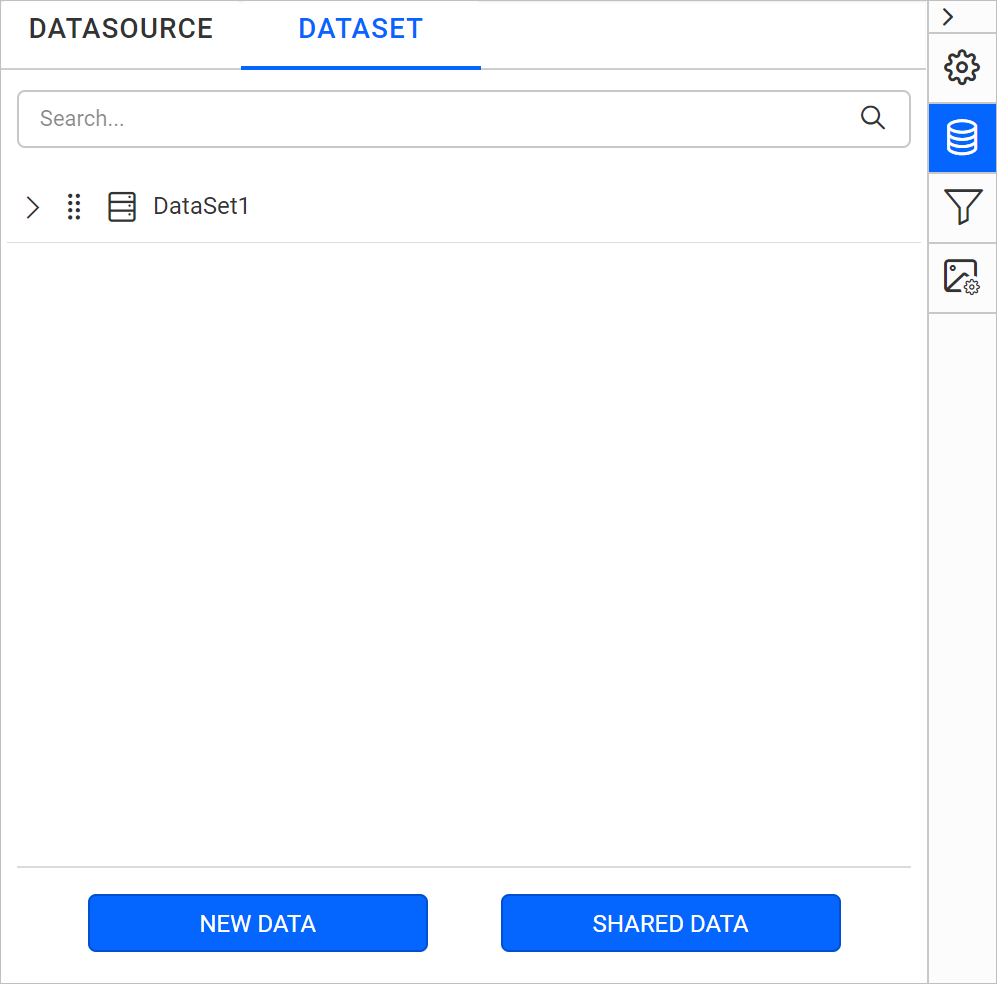This screenshot depicts a software application interface designed for data management and sharing. 

In the upper left corner, there are two selectable tabs labeled in all caps: "DATA SOURCE" (not selected, shown in black text) and "DATA SET" (current selection, shown in blue text with a blue underline). A horizontal dividing line separates these tabs from a search bar below. The search bar contains placeholder text in gray, "search..." accompanied by a magnifying glass icon on the far right. 

Directly beneath the search bar is a drop-down menu indicated by a right-facing triangle (like a bracket). The menu icon consists of a grid with four rows and two columns of dots. Below this icon, there are three rows that appear to be document icons, one of which is labeled "Data Set 1". This section is followed by another horizontal gray dividing line that introduces an expansive empty white space occupying the majority of the image. 

Further down, the white space is bordered by another gray horizontal line, below which lie two action buttons. Both buttons are blue with white text; the left button reads "NEW DATA" and the right button reads "SHARED DATA," both styled in all caps.

The far right edge of the screenshot showcases a narrow vertical column, approximately 5% of the total image width, containing several menu options. This column starts with another right-facing drop-down arrow, followed by a dividing line. Below are four icons: a settings gear (not selected, with a white background), a stack-of-coins-like cylinder (selected, with a blue background), a filtering funnel, and an image icon with an overlaid gear. These icons occupy roughly the top one-third of the vertical space in the column, with the remaining space left blank.